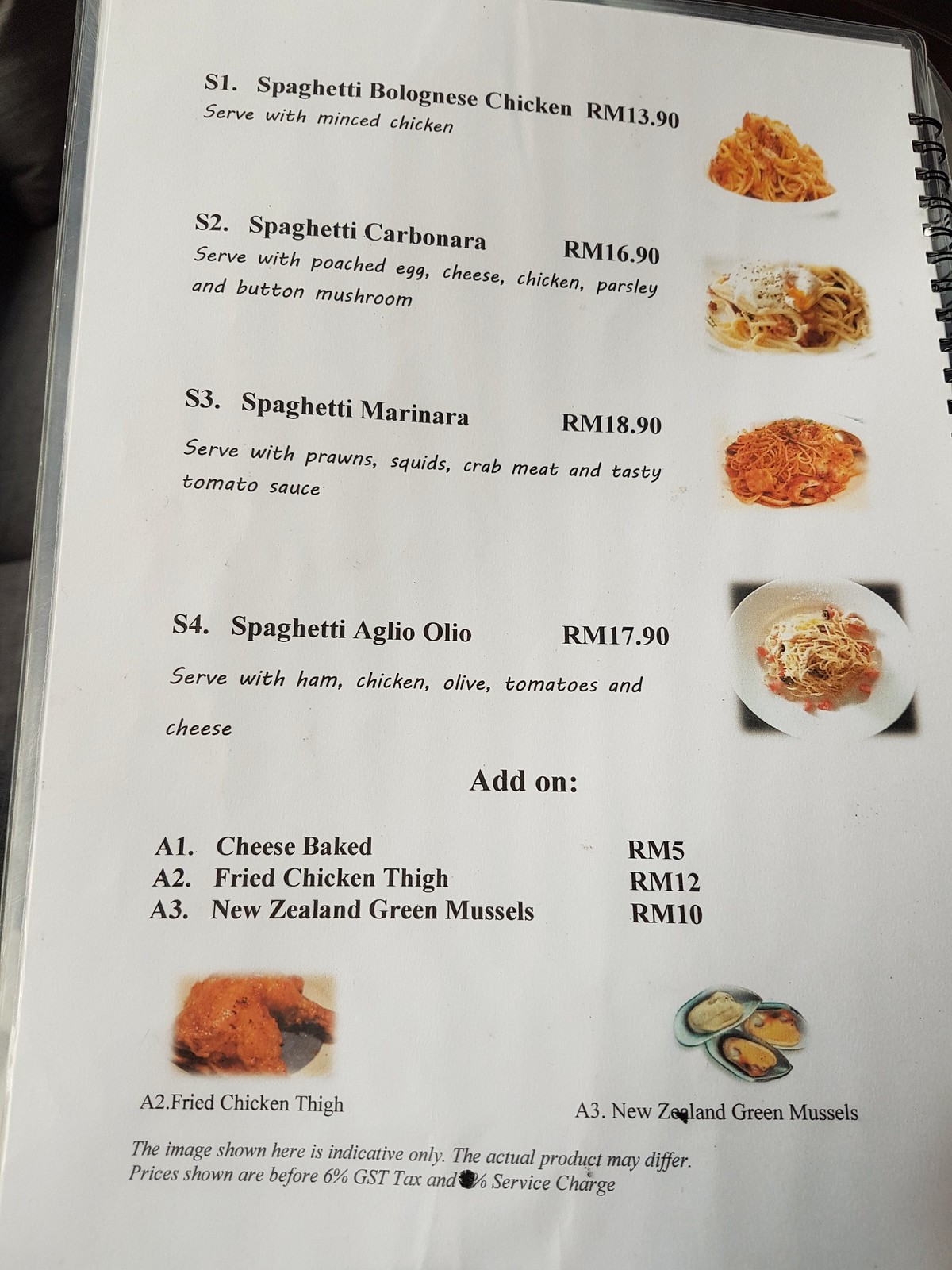### Menu Description

**S1 Spaghetti Bolognese Chicken** - RM 13.90  
Served with minced chicken.  
![Image of Spaghetti Bolognese Chicken]

**S2 Spaghetti Carbonara** - RM 16.90  
Served with poached egg, cheese, chicken, parsley, and button mushrooms.  
![Image of Spaghetti Carbonara]

**S3 Spaghetti Marinara** - RM 18.90  
Served with prawns, squids, crabmeat, and a tasty tomato sauce.  
![Image of Spaghetti Marinara]

**S4 Spaghetti Aglio Olio** - RM 17.90  
Served with ham, chicken, olives, tomatoes, and cheese.  
![Image of Spaghetti Aglio Olio]

### Add-Ons

**A1 Cheese Baked** - RM 5  
**A2 Fried Chicken Thigh** - RM 12  
![Image of Fried Chicken Thigh]

**A3 New Zealand Green Mussels**  
![Image of New Zealand Green Mussels]

**Note:**
- The images shown here are indicative only. The actual product may differ.
- Prices shown are before 6% GST tax and an unspecified percentage service charge (covered by a black dot).
- This menu is presented on a laminated white ring folder.